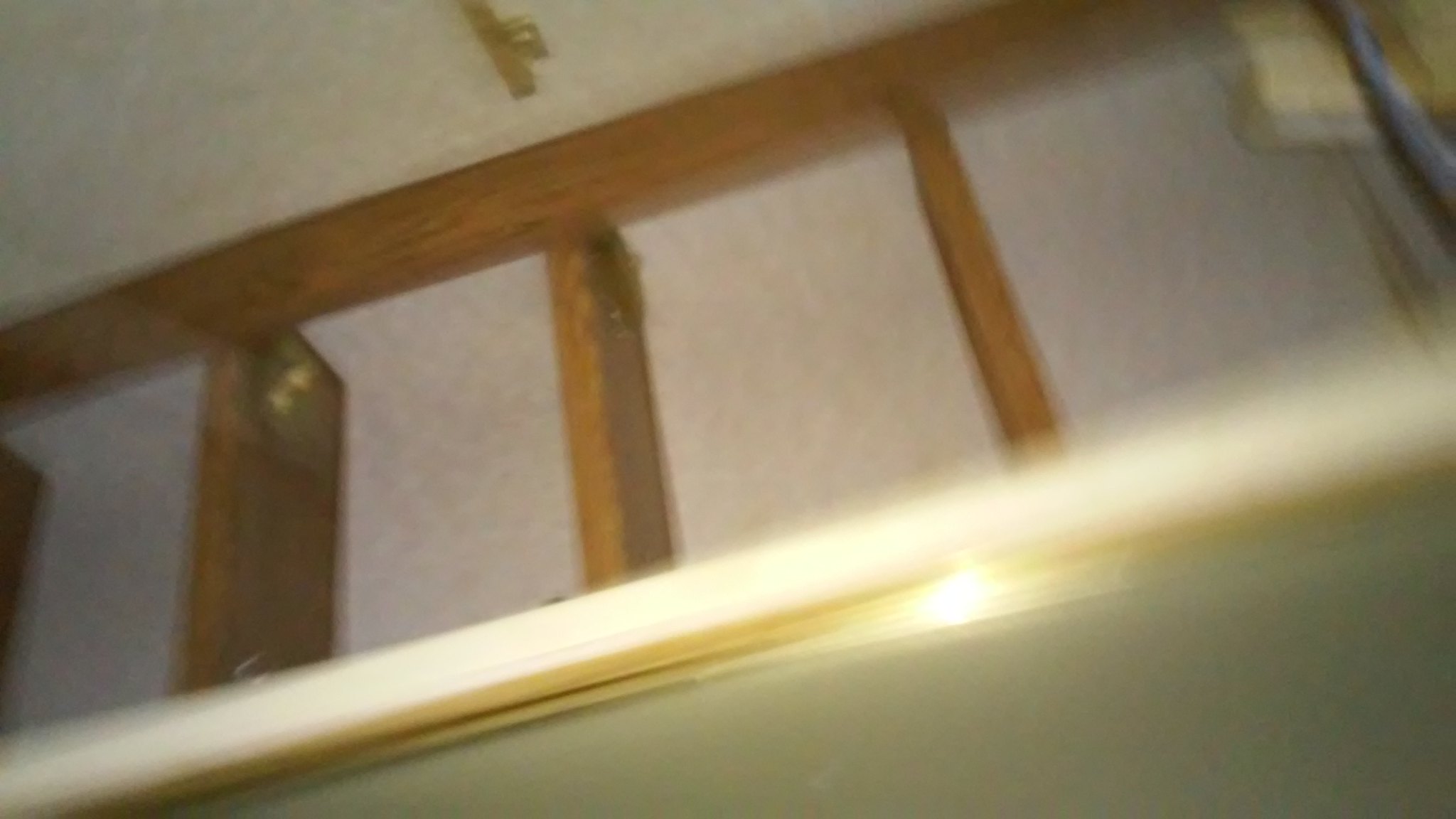A very blurry photograph features a close-up of a wooden structure, which might be an attic ladder or a railing, though the distortion suggests it could be a reflection. The central focus is a wooden formation with horizontal and vertical elements, resembling ladder rungs. These rungs are spaced at intervals: one partially visible on the far left, another in the center, a third on the right, and a final structure towards the top or right end, which is unclear. Above the top piece of wood, another element runs perpendicular; it might be wood, metal, or a lock, suggesting a possible connection to attic stairs. At the bottom, a bright gold rim reflects the camera flash, hinting at a mirror. Below this, a solid painted wall, possibly greenish or grayish, occupies the background. The image is grainy, indicating it was taken in low light conditions.